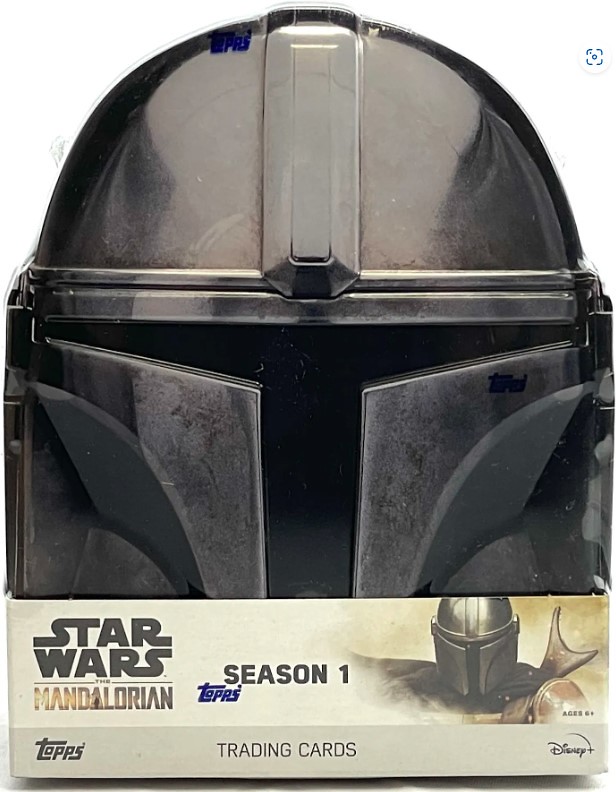This image showcases the front of a Star Wars trading card deck themed around The Mandalorian, specifically Season 1. Dominating the top of the product is an all-black Mandalorian helmet, reminiscent of Boba Fett's, displayed centrally within the image. Encased in plastic, the entire package exudes a sleek and polished finish. Beneath the helmet, a small rectangular label features the "Star Wars" logo on the left, followed by "The Mandalorian" in the distinctive series font. This label continues with the "T.O.P.S." logo on the left and "Season 1 T.O.P.S." in blue font centrally positioned, along with the words "trading cards" below it. In the bottom right corner, the Disney logo is visible, with some small, unreadable text positioned above it. A striking illustration of a Mandalorian character, adorned in a helmet and cape that sway to the left and blend into a white background, further embellishes the bottom section of the packaging. The predominant colors of the image consist of darker hues, including gray, black, beige, tan, brown, and blue, making the overall aesthetic bold and futuristic.